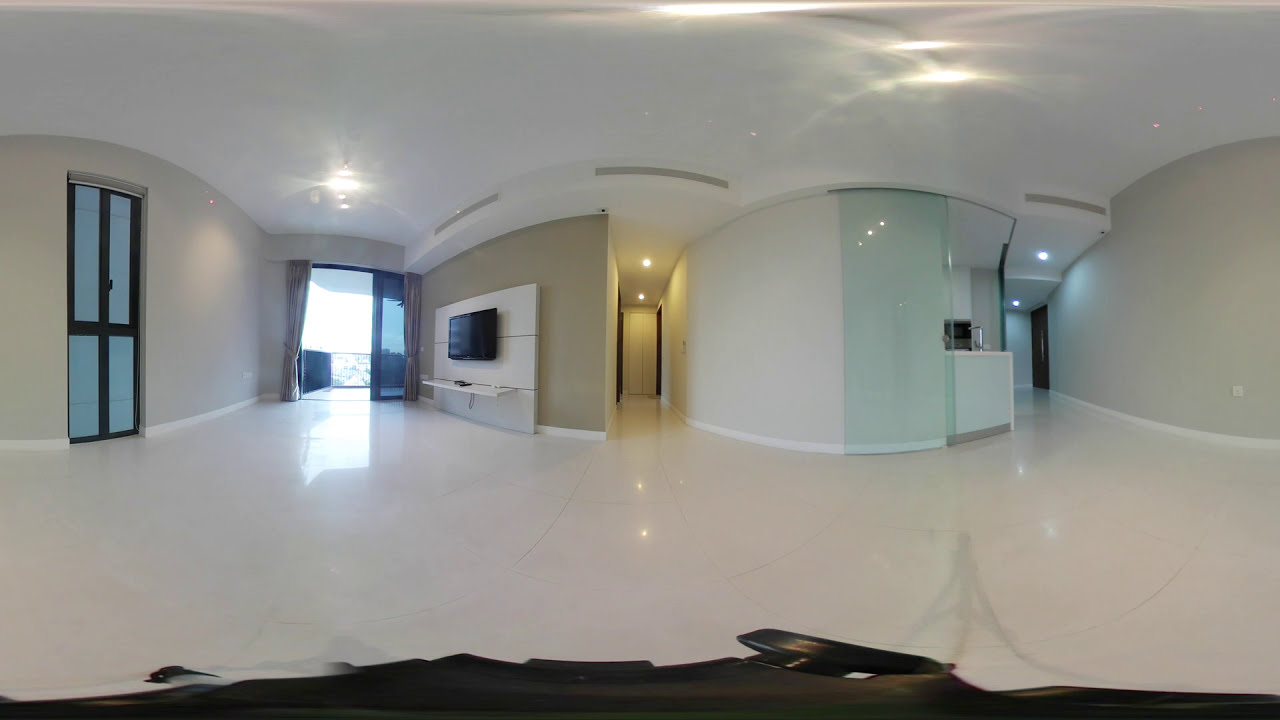The image depicts a meticulously clean and almost sterile indoor environment that appears to be someone's home, though it could easily be mistaken for a hospital due to its spotless nature. Starting from the left, the scene features a doorway along a predominantly white wall with slight touches of beige and the occasional hint of turquoise. Moving rightward, there is an open doorway leading to a balcony, flanked by simple yet elegant curtains. Sunlight streams in from the balcony, illuminating the delicate gray patterns on the white marble floor below. Adjacent to this, a flat-screen TV is mounted on the wall. Continuing further right, another doorway becomes visible, leading into a hallway that presumably connects to the bedrooms. To the right of this hallway, there is a glimpse of a glass-enclosed kitchen area. The room overall features off-white walls, white ceilings, and a few beige accents, completing the minimalist and pristine aesthetic.